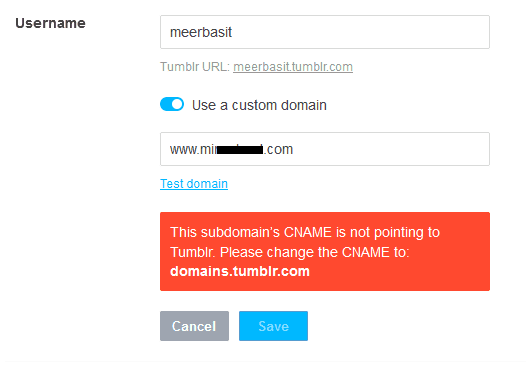**Detailed Description of the Image:**

The image features a user interface on a white background. On the upper left-hand side, there is the word “Username” displayed in dark black font. To the right of this word, there is a white text box containing the text "MEERBASIT" in black font. 

Below this, in grey font, it reads “Tumblr URL”, followed by “name.tumblr.com.” Further down, there is a toggle switch highlighted in blue, indicating it is turned on. Next to the switch, in black font, the text reads “Use a custom domain.”

Beneath this section, there is a search box with the text “www.mi” followed by a blacked-out portion, and then “.com.” Under this, there is blue underlined text that says “Test domain.”

Towards the bottom, an orange-red warning box with white capital letters reads: "This subdomain's CNAME is not pointing to Tumblr. Please change the CNAME to domains.tumblr.com."

Finally, at the very bottom of the interface, there are two blue buttons with white text: the button on the left says “Cancel,” and the button on the right says “Save.”